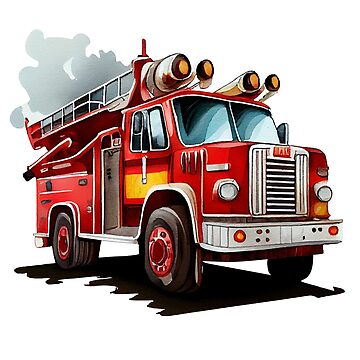This illustration is a detailed cartoon depiction of a vibrant red fire truck in motion, heading to the right. The truck features a prominent silver front grill and bumper adorned with red lights. It has two headlights and a quartet of silver sirens or horns with orange centers situated atop the vehicle above the windshield, which is a blend of black, white, and bluish-gray hues. The fire truck's door exhibits a distinct design: entirely red with a black window, a dark red panel below it, followed by a yellow rectangular stripe. The black wheels are accented with red interior rims. A silver ladder runs along the back top end of the truck, and faint, artistic smoke designs are depicted emanating from the rear. The illustration also includes a reflective black shadow underneath the fire truck, complemented by a background of gray and white smoke. There are no visible occupants inside the vehicle.